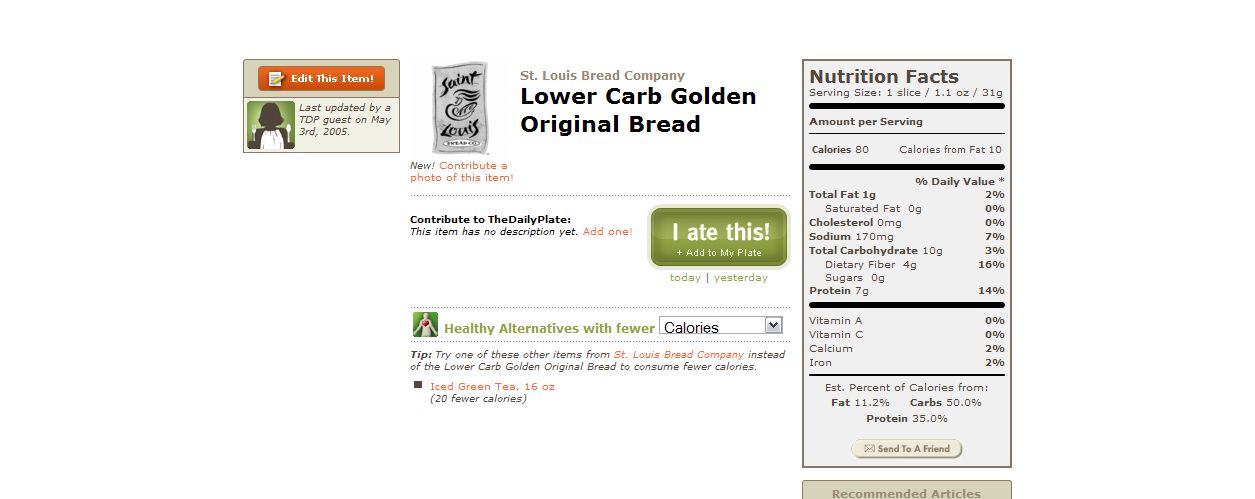This image features a label from a loaf of bread. The label predominantly uses a white background with black script. Centrally positioned on the label is a small green tag that reads "I ate this." To the left of this tag, there is a section with an orange banner at the top that is difficult to read. Below the banner, the text clearly states "Lower Carb Golden Original Bread." This section provides various nutritional facts and figures, though the details are challenging to decipher due to the faint and small print. On the right side of the label, a nutritional information table is present, intended to convey full dietary information typical for a bread product. Additionally, there is a logo displayed on the label, but its details are not legible.